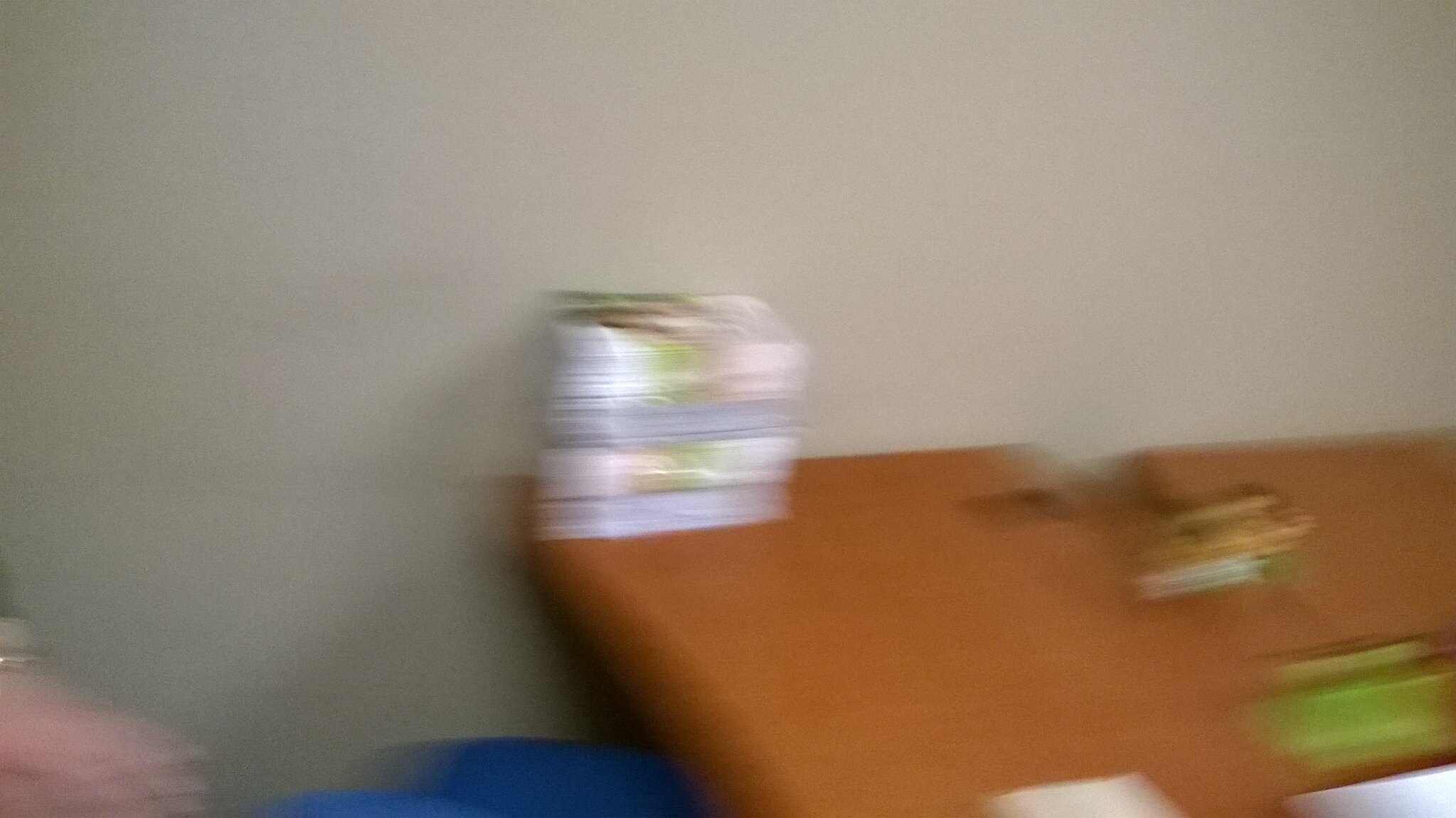The image is an extremely blurry, horizontally rectangular photo showing a segment of a room with an off-white wall. Extending from just below the center-right of the frame and running towards the left side is a reddish-brown wooden table, which makes a 90-degree angle and comes down to the lower center of the frame. The image has significant motion blur, making it difficult to discern specific details, though several objects are visible on the table. These objects, which seem to be shrink-wrapped or perhaps booklets, include hints of white, lime green, and yellow among other indiscernible colors. In the bottom left corner, there is a blur of blue and peach, possibly indicating the presence of a person, with what might be a hand or face showing a tan, skin color, and a hint of an eyeball.